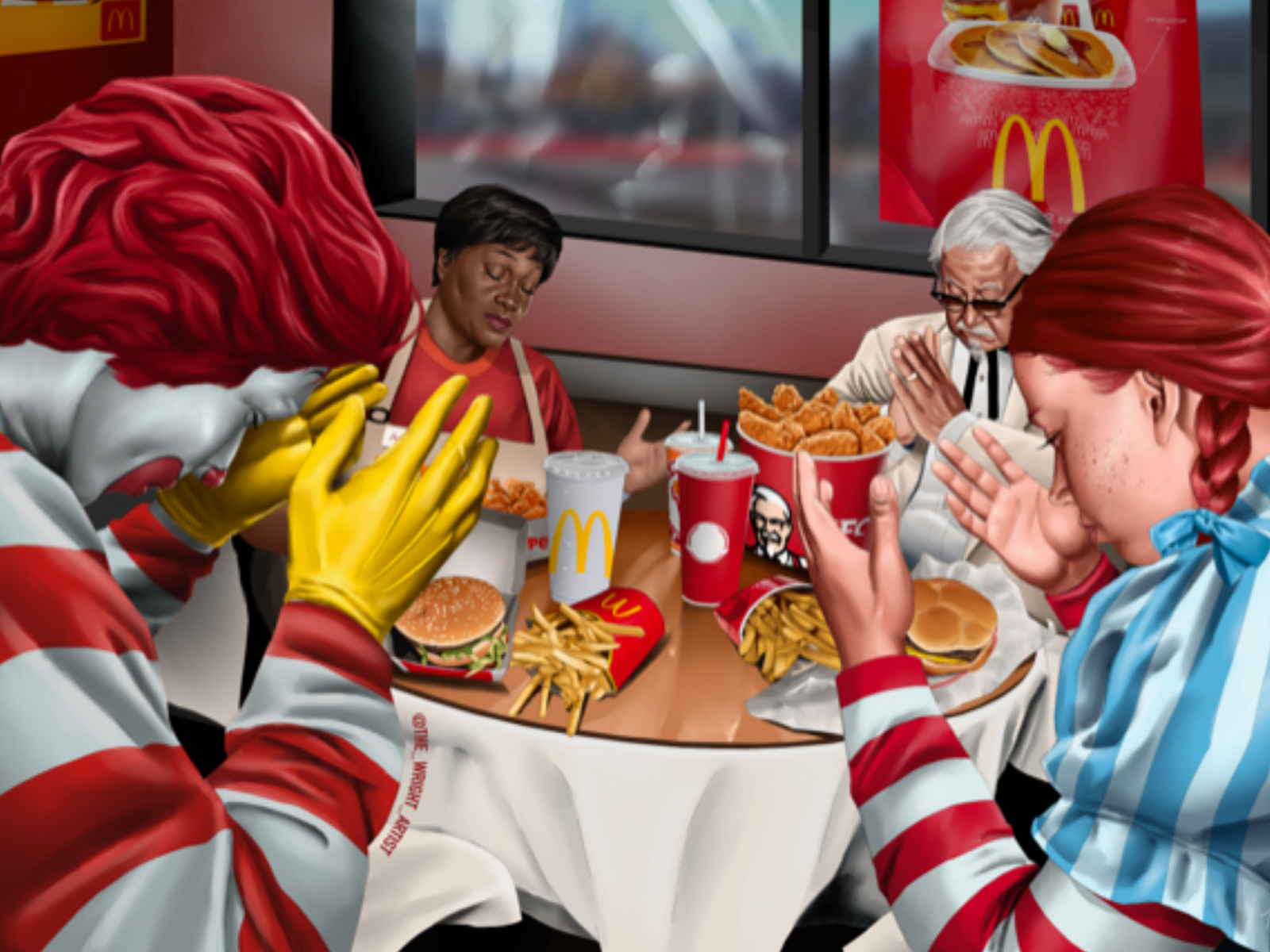In the digital image, four iconic fast food mascots—Ronald McDonald, Wendy from Wendy's, Colonel Sanders from KFC, and the Popeyes lady—are sitting together around a table, presumably in a McDonald's restaurant. The table is laden with their respective branded foods: a Big Mac, french fries, and a McDonald's drink in front of Ronald McDonald; a Wendy's burger, fries, and a drink in front of Wendy; a bucket of KFC chicken before Colonel Sanders, and a box of Popeyes chicken with a drink in front of the Popeyes lady. Ronald McDonald, positioned on the left, has his distinctive red hair, yellow gloves, and red-and-white striped outfit. To his right is Wendy, with her red braided hair, freckled cheeks, and a blue and white striped dress over a red and white striped long-sleeve shirt. Adjacent to Wendy, across the table, is Colonel Sanders, recognizable by his white hair, black sunglasses, white shirt, and black tie, with his hands clasped in prayer. Next to him is the Popeyes lady, distinguished by her short black hair, red shirt, and apron, with her hands raised in a prayerful gesture. The background shows windows and a McDonald's advertisement poster for hotcakes, enhancing the setting's authenticity. Despite their corporate rivalry, the mascots appear unified in a moment of shared grace and prayer before their meal.